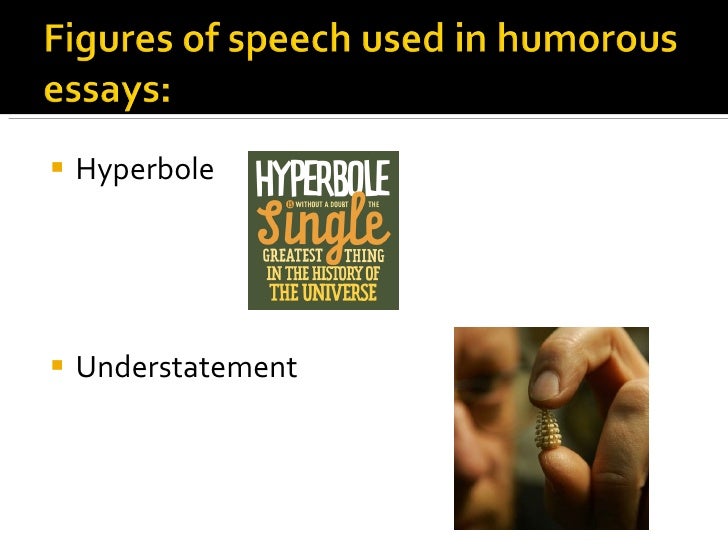**Caption**: 

The image prominently showcases a slide titled **"Figures of Speech Used in Humorous Essays"**, displayed in bold yellow text against a black rectangular bar that spans the top width. Below this title, on a clean white background, are two distinct bullet points in yellow with accompanying black text. 

- The first bullet point reads **"Hyperbole"**. To its right is a book cover in green, adorned with a mix of white, orange, and yellow text. The text on the cover reads: **"Hyperbole: Single Greatest Thing in the History of the Yellow World"**, with "Single Greatest" in yellow, "Thing in the History of the" in orange, and "Hyperbole" in white.
- The second bullet point reads **"Understatement"**. Adjacent to it is an image depicting a male figure wearing thin-wired frame glasses, holding a tiny, spiky, cone-shaped object between his thumb and index finger. The composition of the image focuses on his fingers, making the object the center of attention, while his face remains partially visible and slightly out of focus in the background.

The contrasting colors and distinct images effectively illustrate the playful nature of these figures of speech in humorous writing.